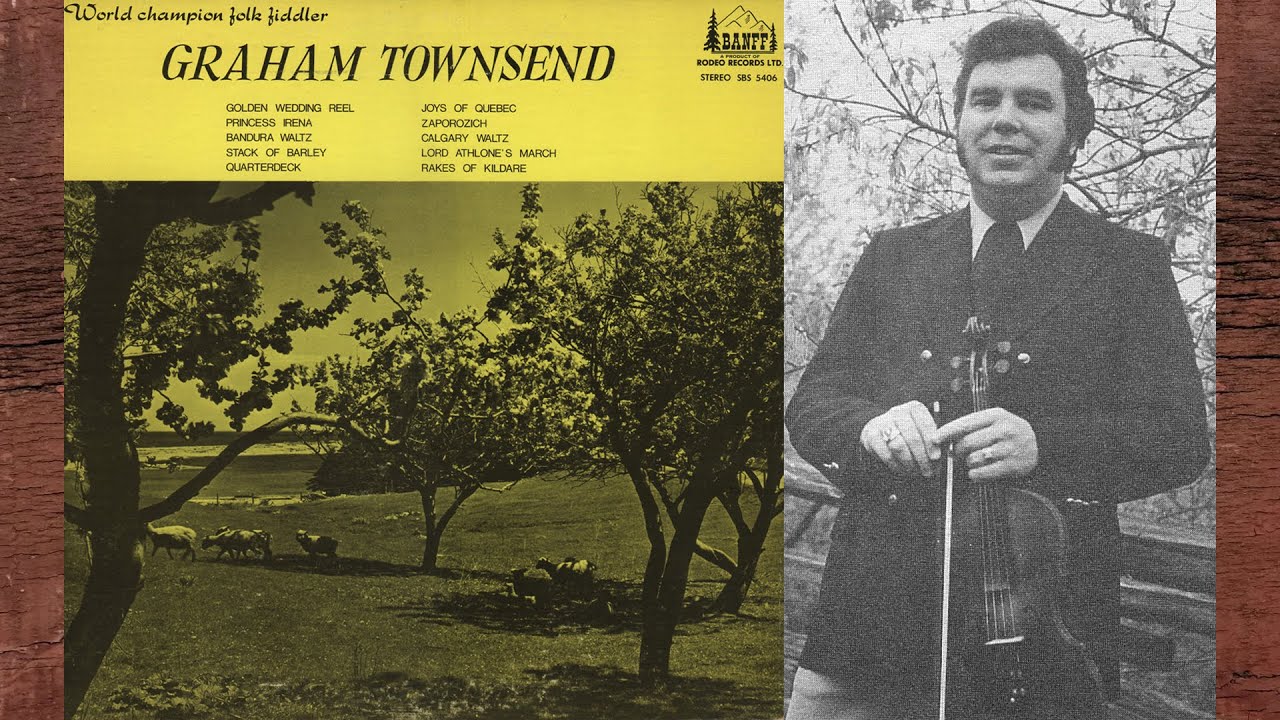The image appears to be an album cover, presented in a horizontal, rectangular format. On the left side, there is a yellow and black-tinted photograph depicting a pastoral scene with trees, a field, and sheep grazing. Above this scene, the text reads "World Champion Folk Fiddler" and "Graham Townsend," followed by a list of song titles including "Golden Wedding Reel," "Princess Vienna," and "Bandura Waltz." Dominating the right side of the cover is a black and white photograph of Graham Townsend himself, a white man with dark hair and long sideburns, reminiscent of the 1960s. He is dressed in a dark suit, with a white button-down shirt and dark tie, and gray slacks. Townsend is holding his fiddle in his left hand and the bow in his right hand, posed against a backdrop that appears to include a tree. The overall design integrates these different elements to prominently feature Townsend and his musical heritage.